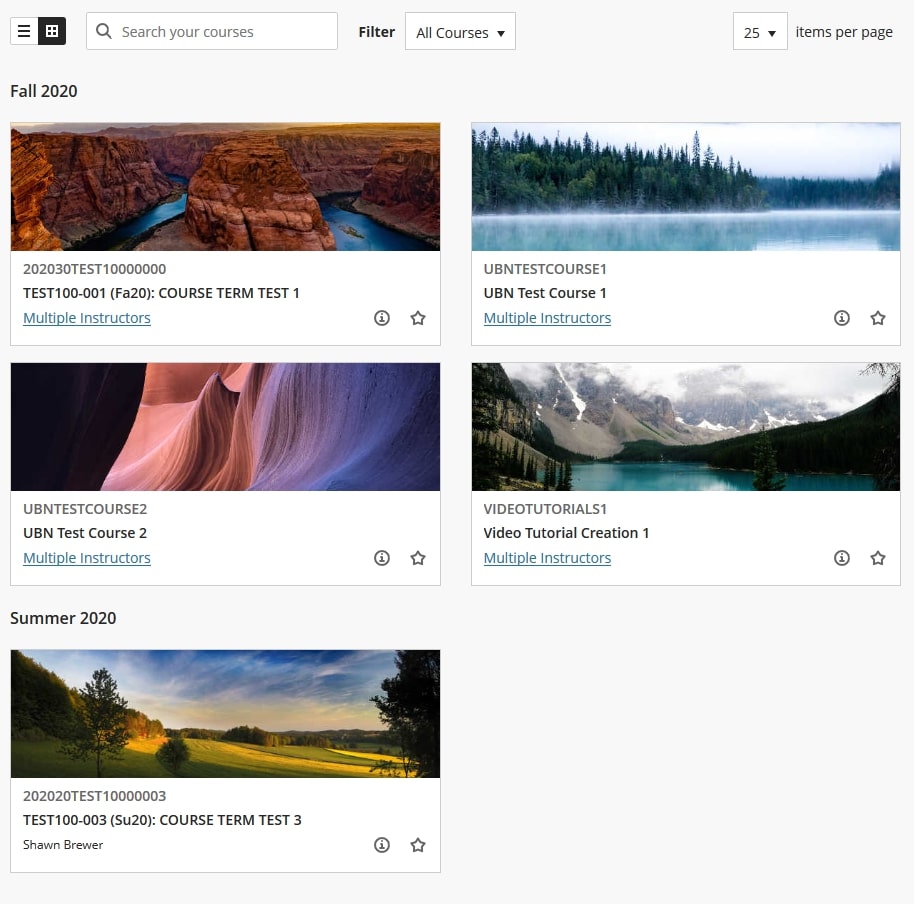Screenshot from a website with a light gray background featuring various interface elements:

At the top left corner, there are two squares side by side – one white with three black horizontal lines stacked on top of each other (representing a menu), and one black with a white square inside containing a cross (likely an icon for a specific feature).

Below these icons, there is a search bar with a white background, a magnifying glass icon, and the placeholder text "Search your courses". To the right of the search bar, there's a "Filter" button in black text (capital F) followed by a drop-down menu labeled "All Courses" on a white background. Further to the right, another drop-down menu displays the number "25" with the label "Items per page".

On the left side, the term "Fall 2020" is printed in black text. Below this header, five course images and details are displayed in a two-column format – three on the left and two on the right.

1. The first course image shows a scenic outdoor view of a mountain range with a river flowing through it. The text below reads "Test 100-001 (FA20 Court)". "Course Term Test One" is detailed in blue hyperlink with "Multiple Instructors".

2. The second course image depicts pink and purple sand dunes, labeled with "UBIN Test Course Two" and associated with "Multiple Instructors".

3. The third course image, titled "Summer 2020", features an outdoor scene with a cloudy sky above a meadow and trees. This course is labeled "Test 100/RA3 Course Term Test Three" and "Sean Brewer". Below that, "UBIN Test Course One" is noted, followed by "Multiple Instructors" as a blue hyperlink.

4. The fourth image, without a detailed description, is labeled "Video Tutorials" and "Video Tutorial Creation One" with "Multiple Instructors".

This detailed layout presents a structured overview of the courses available, complete with visual and textual information to guide users in their selection.